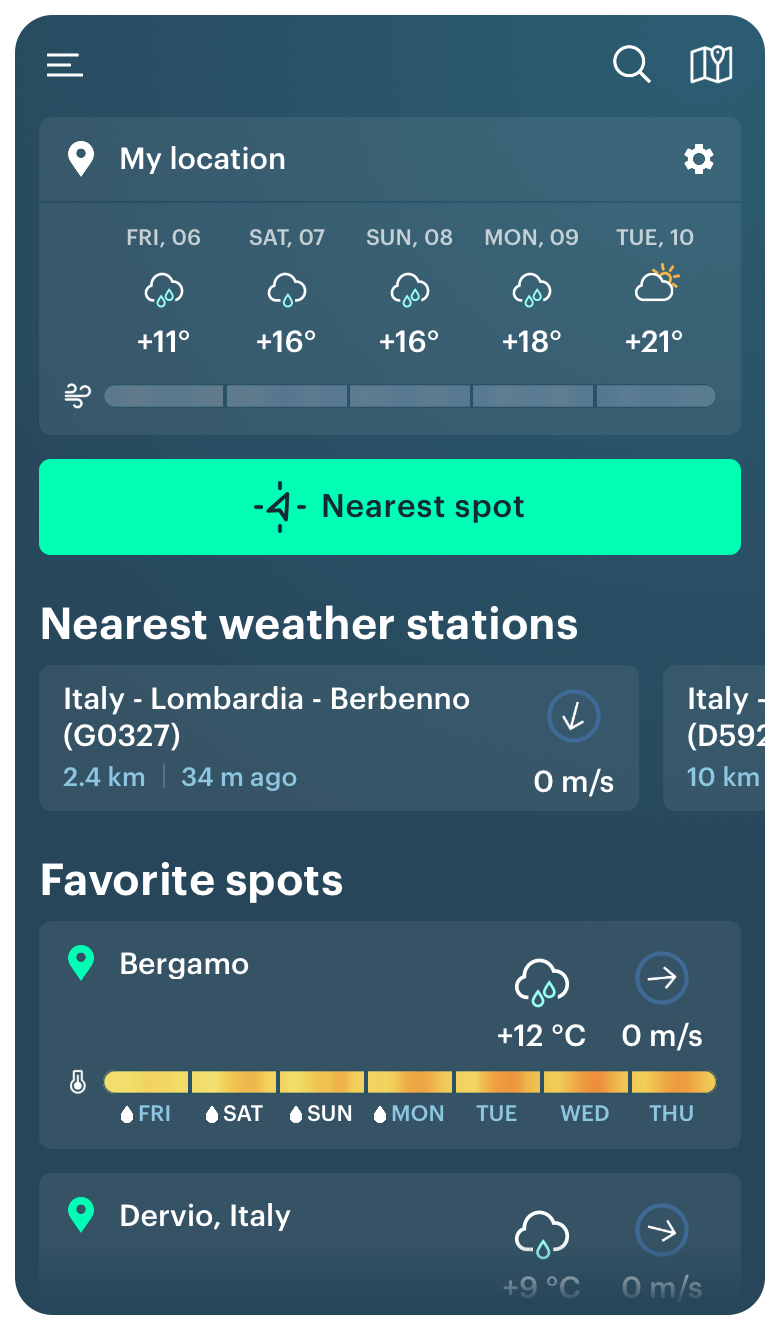This screenshot, captured from a cell phone, features multiple layers of information organized neatly within a user interface. 

At the top, the menu bar on the left side includes options such as a menu icon, a search function, "Sky Glass," and a map icon on the far right. 

Just underneath, a bar displays a location icon labeled "My Location" along with a settings button. 

The main content area features a detailed weather forecast for the next five days, spanning from Friday the 6th to Tuesday the 10th. This forecast indicates a positive trend in temperature. Icons are used to illustrate weather conditions, with a cloud and raindrops symbolizing expected rain, and a cloud partially obscuring the sun indicating varied cloudy conditions by the final day.

Below this, a bar containing a wind icon is present, but it appears to be inactive or without further details.

Centrally positioned, there is a prominent green button with an arrow labeled "Nearest Spot," suggesting an option to select the closest weather location.

Further down, the section titled "Nearest Weather Stations" lists specific stations, including locations in Italy, Lombardia, and Urbino. For each, station identification, distance, the time of the latest update, and current wind speed are provided. To the right side of this section, another choice exists although it is partially obscured or not visible in the screenshot.

The "Favorite Spots" section follows below, starting with a location icon and the city of Bergamo. This area provides a seven-day weather outlook. Another city follows subsequently, offering similar forecast information for future dates. 

Overall, the screenshot presents a comprehensive, multi-functional weather application interface, blending current conditions with forecasts and allowing users to personalize their experience based on location preferences.